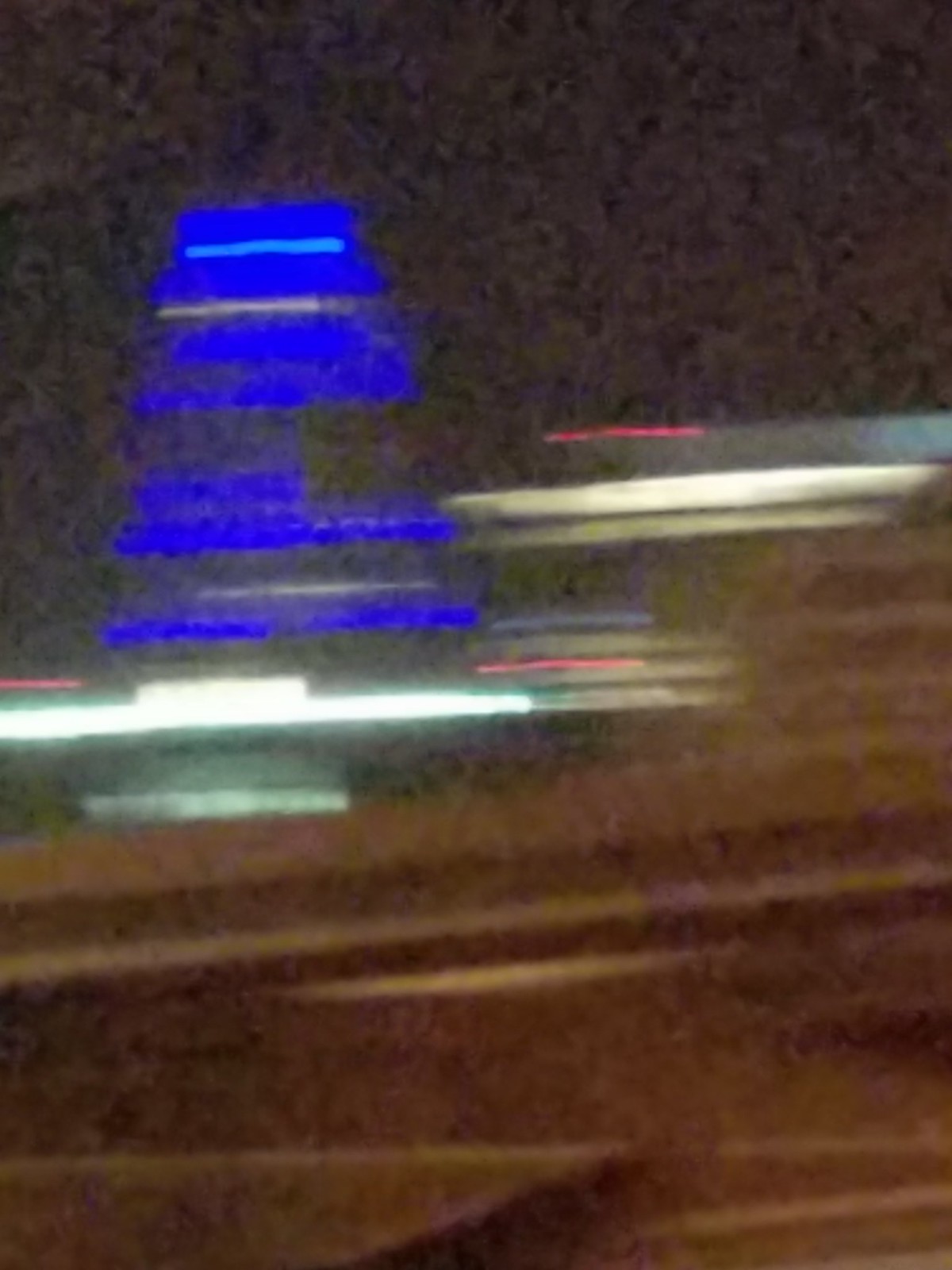This is a color photograph or possibly a painting that employs deliberate blurring and a grainy texture to create an artistic effect. The image features a predominantly gray background in the upper third, marked by lighter and darker textured areas. Moving towards the left, there are several royal blue streaks, which seem more likely to indicate brush strokes from a painting. On the right side, the streaks transition into silvery and grayish white lines, adding further complexity. Below these, additional streaks in white and silver continue the layered effect. In the bottom third of the image, vertical shades of brown suggest the appearance of a hardwood floor, creating a multi-dimensional and thoughtfully crafted visual experience.